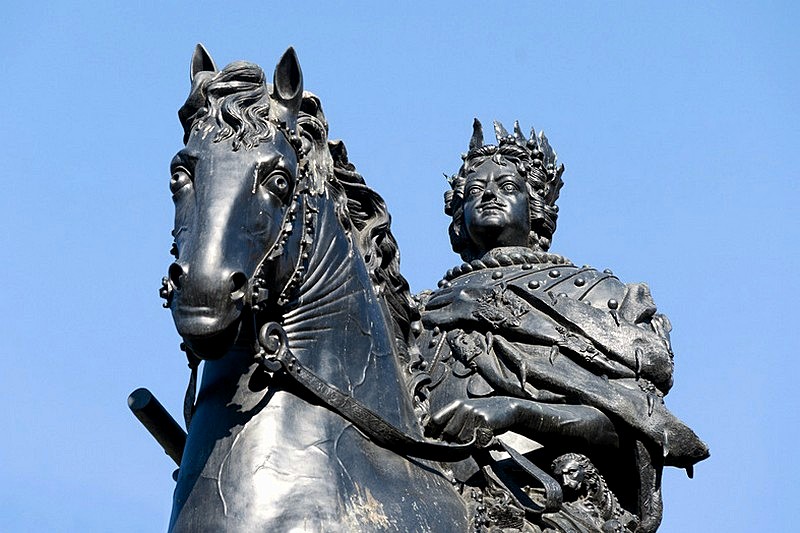The photograph depicts the upper portion of a detailed statue of a man, likely a king or a warrior, astride a horse. The statue, cast in a dark, silvery metal, showcases the rider wearing a crown atop his curly, billowing hair, and armor beneath a cloak adorned with nubs. He holds the reins in his left hand, and a large ring is noticeable on his pinky finger. The rider's thin mustache and regal appearance further emphasize his royal status. The horse, positioned to the left, has a finely sculpted head with a long nose, wavy mane, and pointy ears. The horse's neck veins are intricately depicted, and its eyes are carved with holes where the pupils would be. The background features a clear, blue sky, indicating that the statue is situated outdoors. A sword's hilt is slightly visible to the right of the rider, adding to the elaborate and historical nature of the statue.